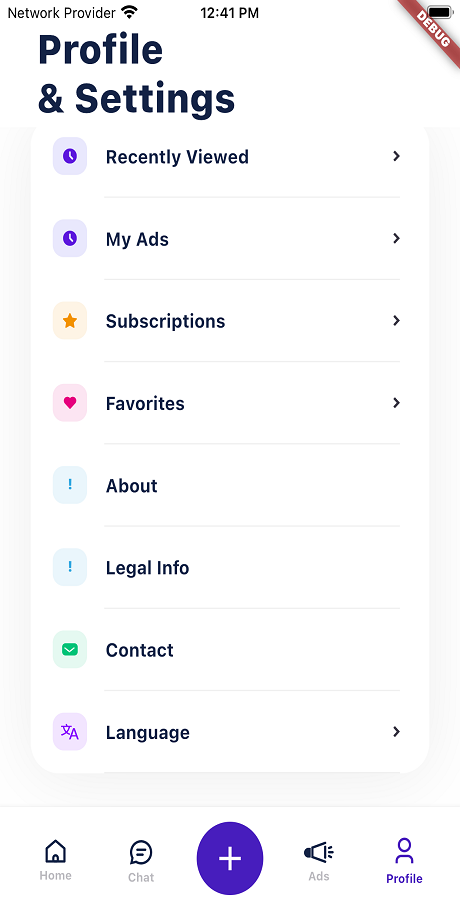This screenshot showcases a mock-up of a "Profile and Settings" page on a cell phone. At the top right, a red banner diagonally labeled "DEBUG" stands out. On the top left, "Network Provider" is indicated in black text, followed by a Wi-Fi icon, suggesting the context is part of a tutorial. Just beneath, the title "Profile and Settings" is prominently displayed in large black font. The page is organized into various categories listed vertically.

1. **Recently Viewed** - An arrow points to the right for expansion.
2. **My Ads** - Also expandable, indicated by a right-facing arrow.
3. **Subscriptions** - Includes an arrow for expansion.
4. **Favorites** - Comes with an arrow suggesting further options.
5. **About**
6. **Info**
7. **Contact**
8. **Language** - Expandable with a right-facing arrow.

At the bottom of the screenshot, a navigation bar features icons for:
1. **Home**
2. **Chat**
3. **A purple circle with a plus sign** centralized in the middle.
4. **Ads** - represented by a megaphone icon.
5. **Profile** 

The design and structure imply a user-friendly interface aimed at managing different aspects of the profile and settings efficiently.